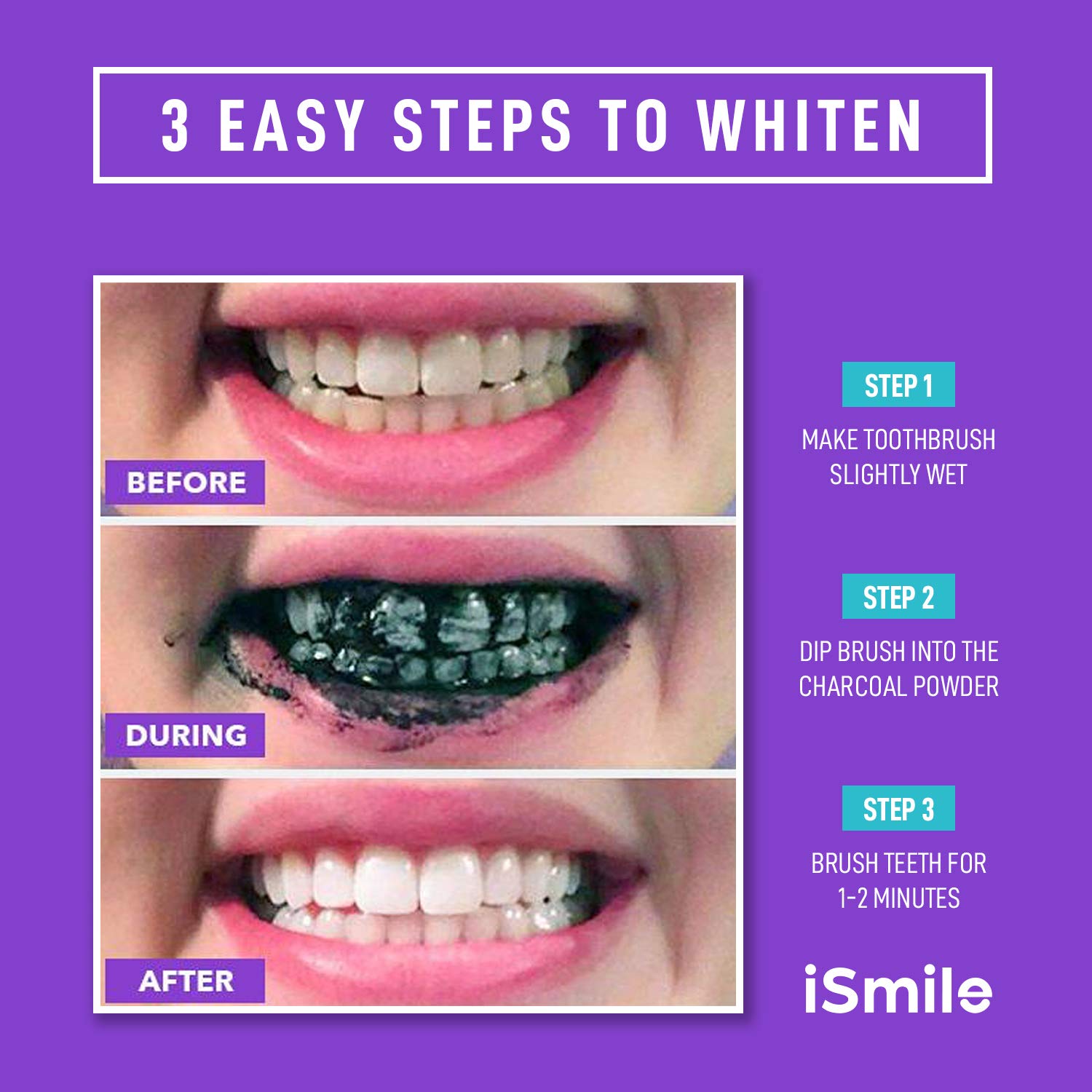The image is an advertisement for a product called iSmile, designed to whiten teeth using charcoal powder. The background is bright purple, and at the top of the advertisement, bold white text with a white box around it reads, "THREE EASY STEPS TO WHITEN." Beneath this, three sequential pictures display a person’s mouth, each demonstrating a different stage in the whitening process. The first picture, labeled "BEFORE," shows the person’s slightly yellow teeth. The second picture, labeled "DURING," depicts the person's teeth covered in a black charcoal powder, smeared from brushing. The final picture, labeled "AFTER," reveals noticeably whiter teeth. Accompanying these images are captions outlining the steps: "Step one: Make toothbrush slightly wet," "Step two: Dip brush into the charcoal powder," and "Step three: Brush teeth for one to two minutes." In the bottom right corner of the advertisement, the product name "iSmile" is prominently displayed.